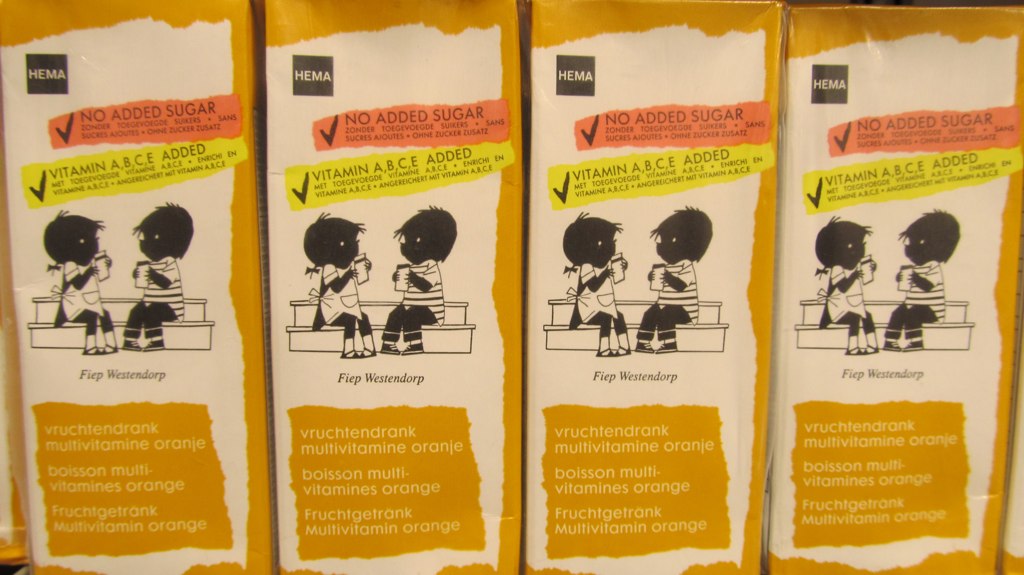The image depicts various sides of a carton, likely containing orange juice. One side of the carton prominently features an illustration of two dark-skinned children sitting on bleachers, enjoying a beverage. The carton proudly advertises "No Added Sugar" and lists the vitamins it contains, including Vitamins A, B, C, and E, notably omitting Vitamin D. The branding includes the term "Multivitamin Orange" in multiple languages, emphasizing the fortified nature of the beverage.